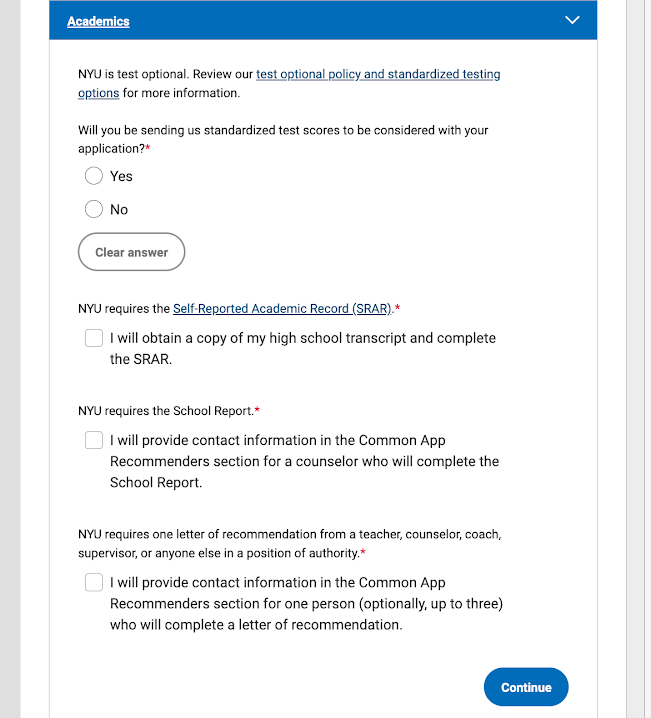A screenshot of an NYU admissions webpage on a white background features a structured mixture of black, white, and blue text. The top of the page displays a blue navigation bar with "Academics" in white font, accompanied by a white pull-down arrow. 

Below, prominently in black and blue text, the page reads, "NYU is test optional." It elaborates further with details in black and blue fonts: "Review our test-optional policy and standardized testing options. For more information, will you be sending us standardized test scores to be considered with your application?" A red asterisk marks this important question, with response options "Yes" and "No" in white circles, neither of which is selected. There is also a "Clear Answer" box available for users to deselect their choices.

The text continues, noting that "NYU requires the Self-Reported Academic Record (SRAR)" with a red asterisk for emphasis. The statement below in black reads, "I will obtain a copy of my high school transcript and complete the SRAR," accompanied by an unchecked white box.

Further down, the page specifies that "NYU requires the school report" (red asterisk). The accompanying text indicates, "I will provide contact information in the Common App recommenders section for a counselor who will complete the school report," featuring another unchecked white box.

Additionally, the requirements include "one letter of recommendation from a teacher, counselor, coach, supervisor, or anyone else in a position of authority," again marked by a red asterisk. The corresponding text states, "I will provide contact information in the Common App recommenders section for one person (optionally up to three) who will complete a letter of recommendation," with another unchecked white box.

Finally, at the bottom of the page is a blue box with "Continue" written in white font, urging applicants to proceed with the application process.